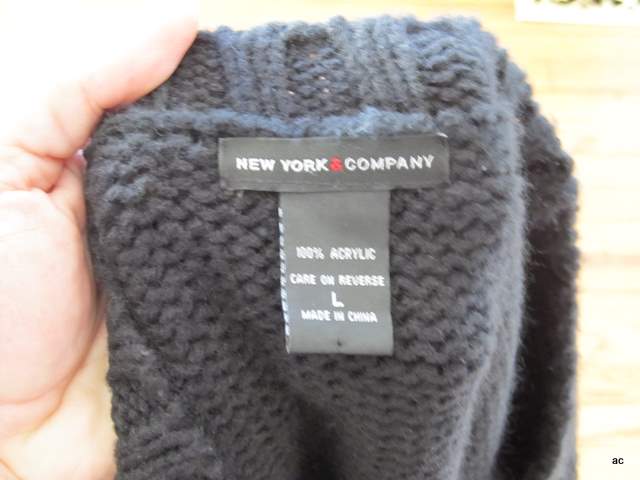This color photo captures a close-up view of a knitted sweater's tag. The sweater, in a navy blue or dark blue hue, features some mild fuzz and pilling but remains in generally good condition. Prominently featured is a black label with white lettering that reads "New York and Company," with a red ampersand. Below this, a vertical tag in white text states "100% acrylic, care on reverse, L, made in China." A left hand with a light skin tone is holding up the sweater, positioned on the left side of the image. The background reveals a brownish hardwood floor on the right, with some light-colored wood paneling barely visible at the top. The photo appears slightly blurry and overexposed, particularly around the hand, which is washed out due to the lighting.